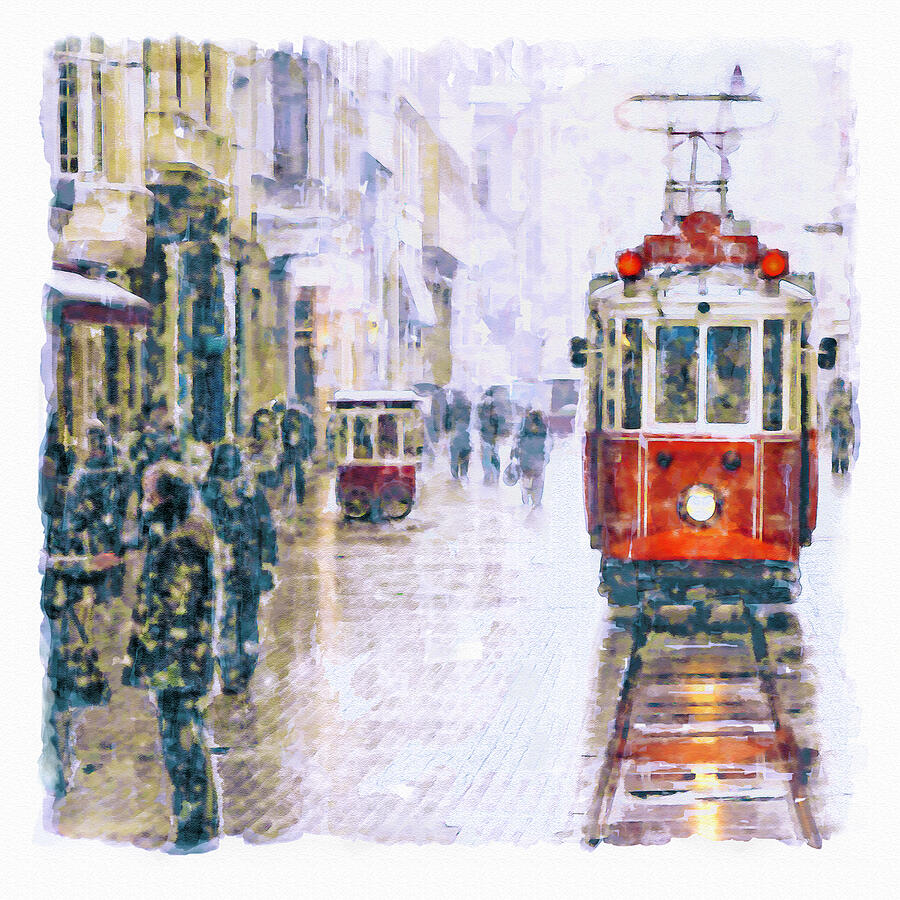The painting depicts a bustling city street, possibly in San Francisco, rendered in an impressionistic style that leaves the figures and their attire somewhat blurry and indistinct. The focal point is a red and white tram or streetcar traveling towards the viewer on grayish-brown tracks. The scene is accentuated by a wintry atmosphere, with snow falling and accumulating on the ground, suggesting a chilly day nearing nighttime, as indicated by the streetcar’s illuminated light. To the left of the streetcar, there are several older style buildings, likely connected or adjacent to one another, and a street cart that appears to be selling goods. People are scattered throughout, bundled up in winter clothing like puffer jackets, scarves, and hats, engaged in conversation or simply moving along the street. The overall imagery evokes a sense of timeless urban life brimming with activity amidst a cold, snowy day.